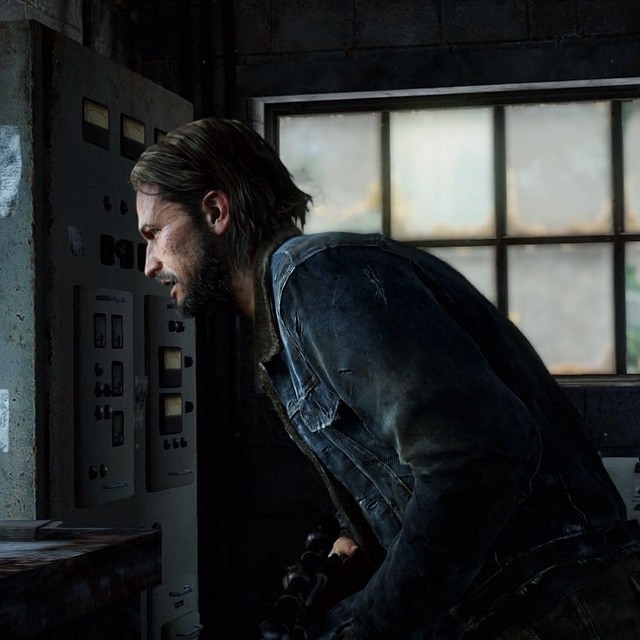A tense movie scene unfolds in a dimly lit room dominated by an industrial aesthetic. A frosted window, divided into individual panels by metallic strips, forms the backdrop, obscuring any view of the outside world. To the left of the window, a complex control panel bristling with buttons and meters is mounted on the wall. Below this panel sits a cluttered desk illuminated by a faint glow, possibly from a computer screen or another light source. In front of the desk stands a rugged man, leaning forward intently as he scrutinizes something on the desk. His right hand grips a gun, adding a layer of danger to the atmosphere. Clad in a worn denim jacket, with medium-length hair framing his bearded face, he exudes a gritty determination, his mustache barely concealing a look of intense focus.